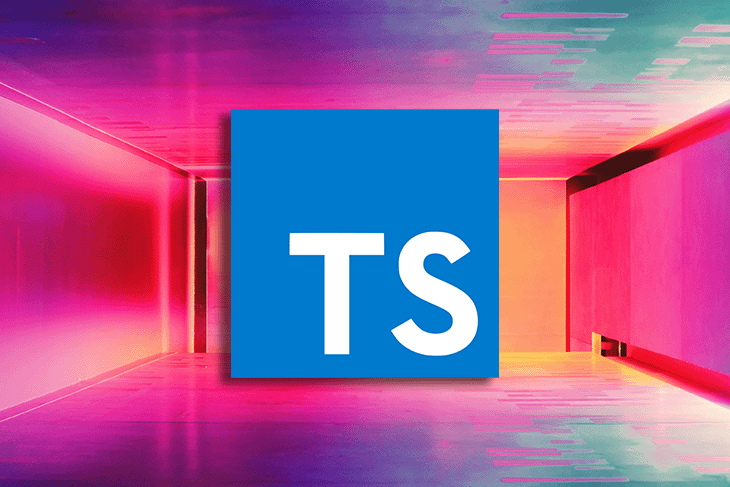This is a computerized drawing, possibly a logo or snippet from a website, featuring a distinctive design. Central to the image is a blue square with a subtle light shading. Positioned in the lower right corner of this square is the bold, white capitalized text "TS." The square appears to float in the middle of a room with a low ceiling, no visible windows, and no identifying features like furniture or TV. The room's walls, floor, and ceiling are rendered in a mix of colors—pink, greenish, purplish, and bluish—giving it a modern, somewhat futuristic atmosphere. Notably, the room includes two openings: a horizontal slit on the floor of the right wall, and a vertical slit running from the floor to the ceiling on the far left wall. There are no people or annotations within the image, adding to its abstract and intriguing quality.